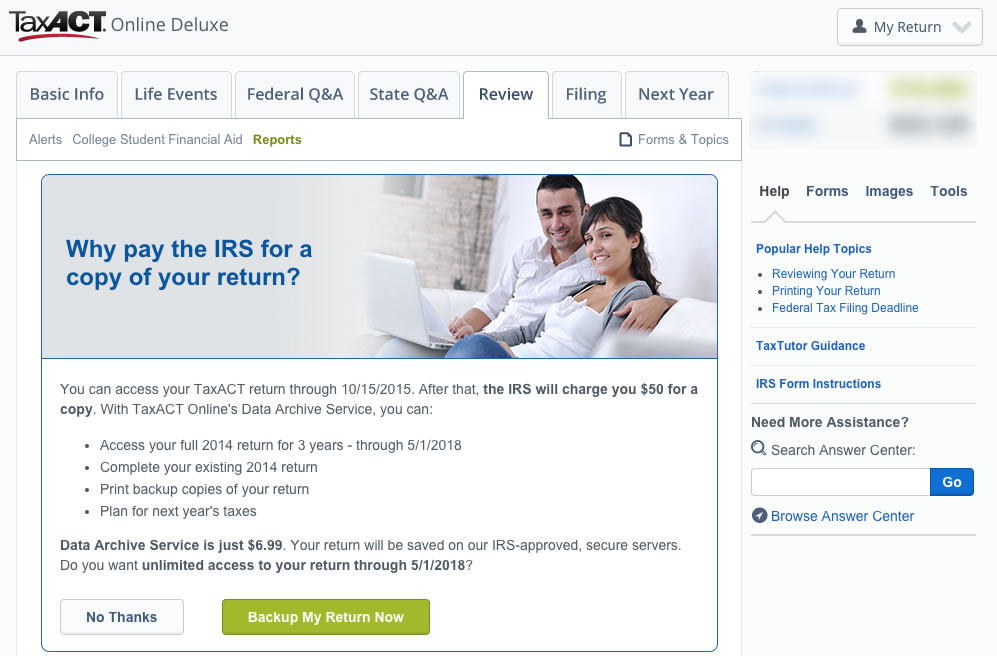The image depicts the TaxAct website interface. The background is predominantly white, with the TaxAct logo prominently displayed at the top. The logo features "TAX" in regular black letters, while "ACT" is in bold capital letters, accompanied by a distinctive red curved line underneath. To the far right of this toolbar is a drop-down menu labeled "MY RETURN."

The central part of the image is occupied by a primary menu laid out in tab style. This menu includes the following categories: BASIC INFO, LIFE EVENTS, FEDERAL Q&A, STATE, REVIEW (which is the currently active tab), FILING, and NEXT YEAR. Directly beneath this is a sub-menu specific to the REVIEW tab, listing options such as ALERTS, COST, STUDENT FINANCIAL AID REPORTS, FORMS, and TOPICS.

Below the main menu, there appears to be an advertisement featuring a smiling couple using a laptop. The ad highlights that users can request a copy of their return until a specified date, with additional details outlined in a paragraph. It also mentions an optional special service available for $7, with options to select "NO THANKS" or to go back.

On the right side of the image, there is a smaller box containing another menu with items labeled HELP, FORMS, IMAGES, and TOOLS. Above this menu, some text is blurred out, likely indicating personal information. At the bottom of this box, users can choose various HELP TOPICS or utilize the SEARCH function for further assistance.